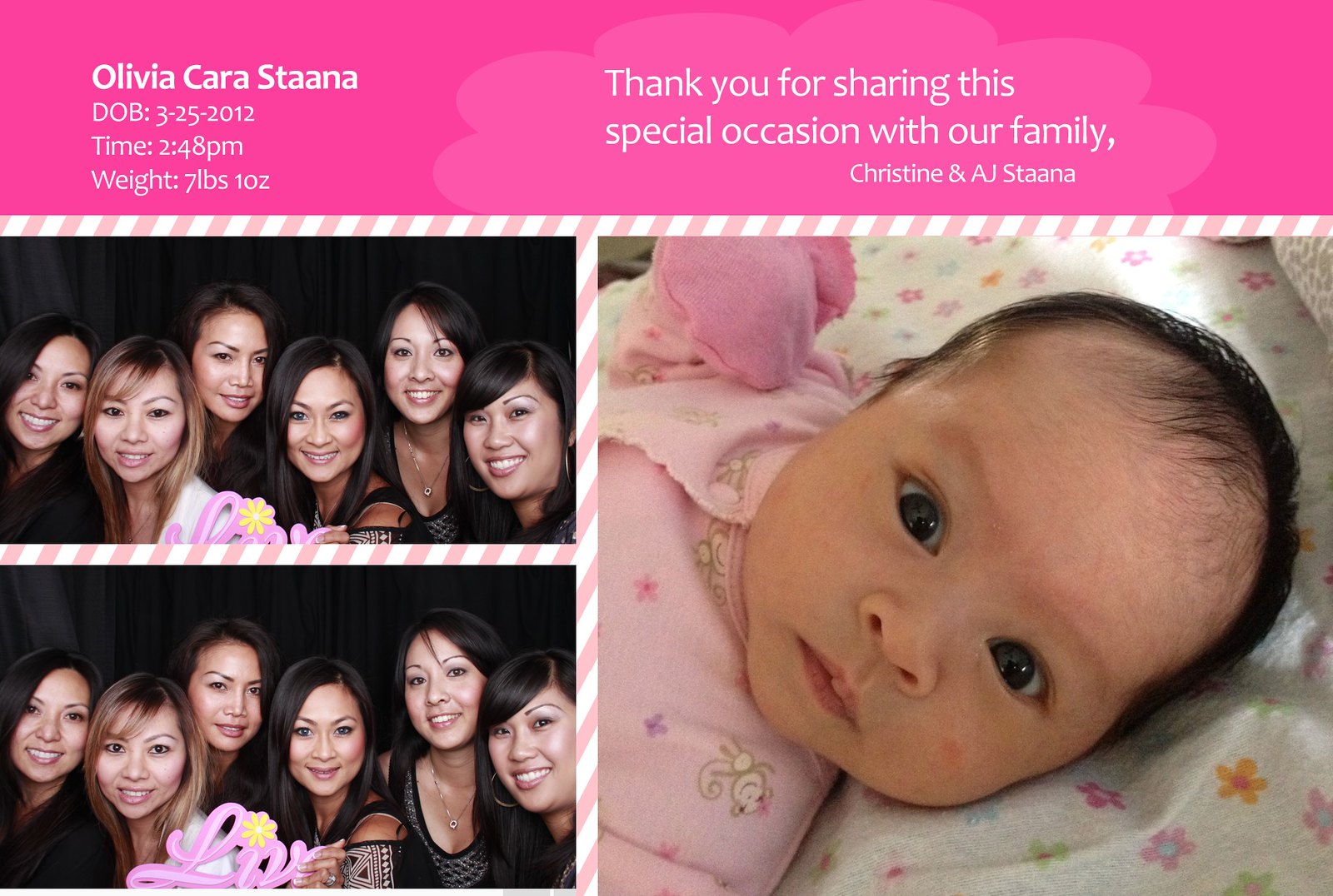The image is a detailed invitation or announcement with text and photographs. At the top, a pink horizontal strip features text in white, which reads: "Olivia Cara Stana, DOB 3-25-2012, Time 2:48 PM, Weight 7 lbs 1 oz. Thank you for sharing this special occasion with our family, Christine and AJ Stana." Below this strip, there are three photographs. On the right half, there is a square image of a young Asian baby with black hair, staring at the camera from a white crib. She is dressed in a pink pajama top adorned with little brown monkeys and is wearing a pink mitten, possibly to prevent her from scratching her face. On the left half are two similar group photos, one on top of the other, depicting five Asian women with long black hair and makeup, posing in front of a black curtain. Their faces and upper bodies are visible, and they are smiling at the camera.